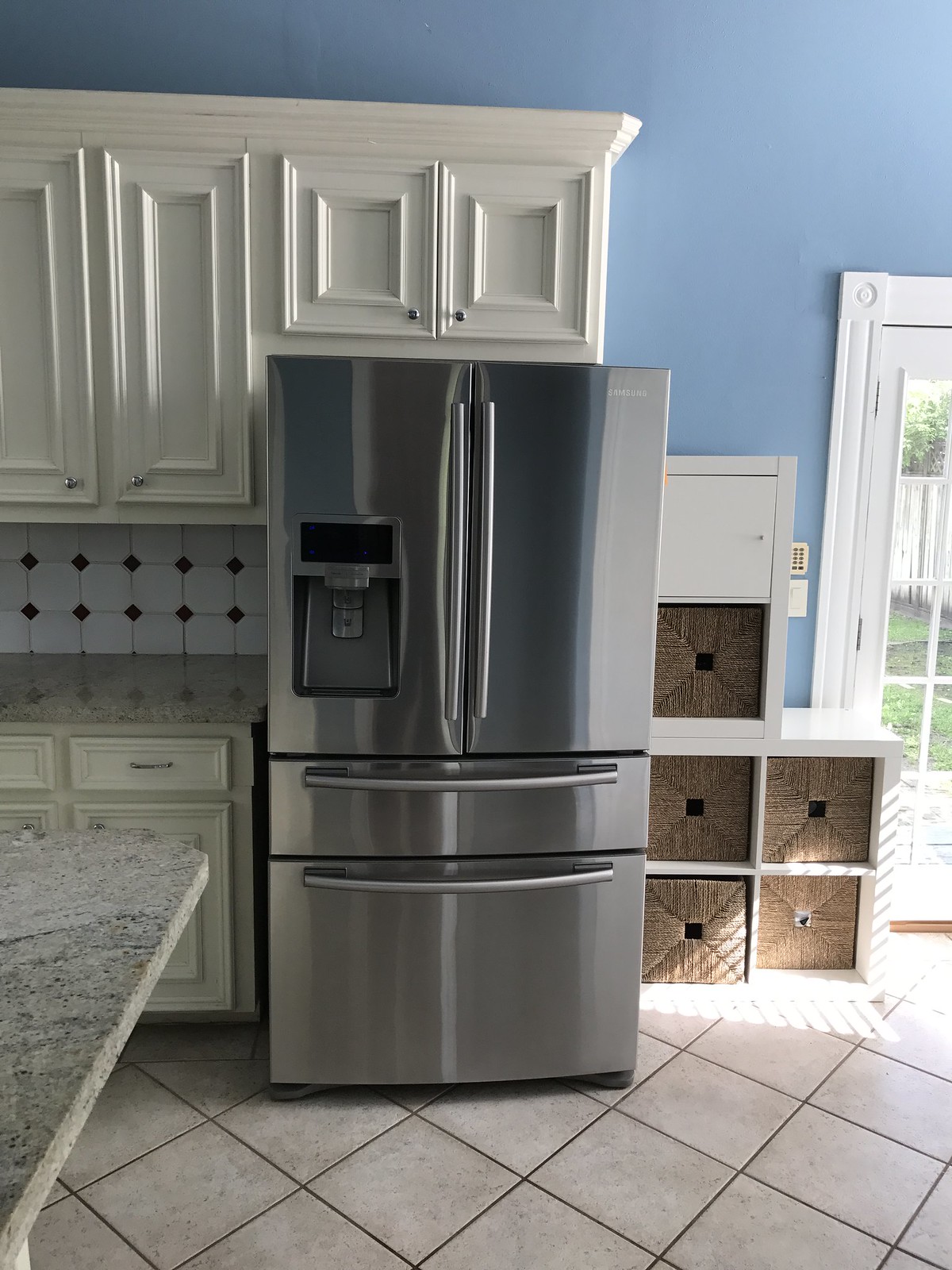The image depicts a sleek, stainless steel refrigerator centrally placed in a starkly empty kitchen, which appears to be relatively new. The refrigerator features double doors at the top, with an ice and water dispenser on the left door and a digital display. Below the double doors is a shallow drawer, about a foot high, followed by a large bottom drawer designed as a freezer. The entire appliance is perfectly nestled under white cabinets. The surrounding cabinetry includes two long doors on the left, with two smaller doors above the refrigerator. 

Directly to the left, the wall is adorned with a pattern of white tiles bordered by black tiles arranged in a diamond shape, extending to a grayish-brown marble countertop. This countertop continues underneath, hosting a stack of drawers and more cabinets. The flooring is composed of light off-white beige square tiles with darker grout lines.

To the refrigerator's right, there's a white shelving unit featuring multiple slots, with wicker baskets fitted into these slots. Some baskets are slightly misaligned, with one apparently broken or pushed back unevenly. Adjacent to this unit stands a glass-paneled door, framed in white, leading to an outdoor view showcasing green grass and trees. The kitchen exudes a clean, uncluttered ambiance, with creamy, off-white cabinets, and countertops that combine shades of gray, black, and white.